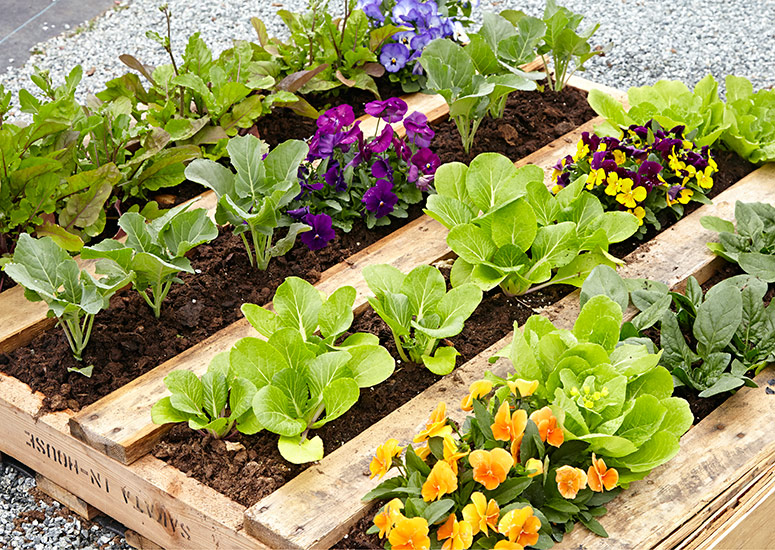This is a color photograph capturing a creative planter made from a wooden pallet, set horizontally on a gray gravel surface. The pallet, which is natural raw wood and somewhat worn, has been modified by removing several slats to make sections of rich, dark brown soil for planting. Each row within the pallet houses a variety of plants and vibrant flowers, arranged in neat, well-cared-for rows. Starting from the left, the first row is predominantly green plants, featuring a bluish flowering plant at the end. The next row has similar green foliage intermixed with purple and green plants, and a striking purple flower in the center. The following row showcases green plants with a beautiful combination of purple and yellow flowers towards the end. The final row contains a combination of orange and yellow flowers alongside additional green plants. The bright and colorful blooms of purple petunias, yellow and orange impatiens, and other mixed flowers stand out against the earthy tones of the soil and wood. The edges of the photo display the gravel and a small glimpse of a road in the top left corner. There are some indistinct letters on the side of the pallet, adding a subtle yet mysterious detail to the scene.